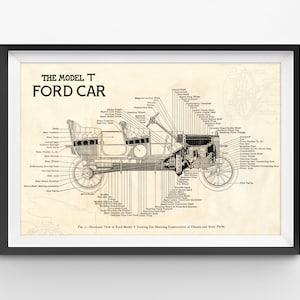The image depicts a detailed design blueprint of the Model T Ford car presented in a black-framed poster. The frame features a thin light blue inner border surrounding the central white section where the blueprint is sketched. The schematic, rendered in black and white with a vintage brownish tone, shows a side view of the car, oriented with the front end to the right and the back to the left. The design highlights the positioning of the front and back seats, the front-end, and the two wheel outlines with spokes. Multiple lines extend from various car parts, connecting to small, hard-to-read labels that likely describe each component. The background appears yellowish, adding to the aged look of the image, and the poster casts a visible shadow, indicating it is mounted on a wall.